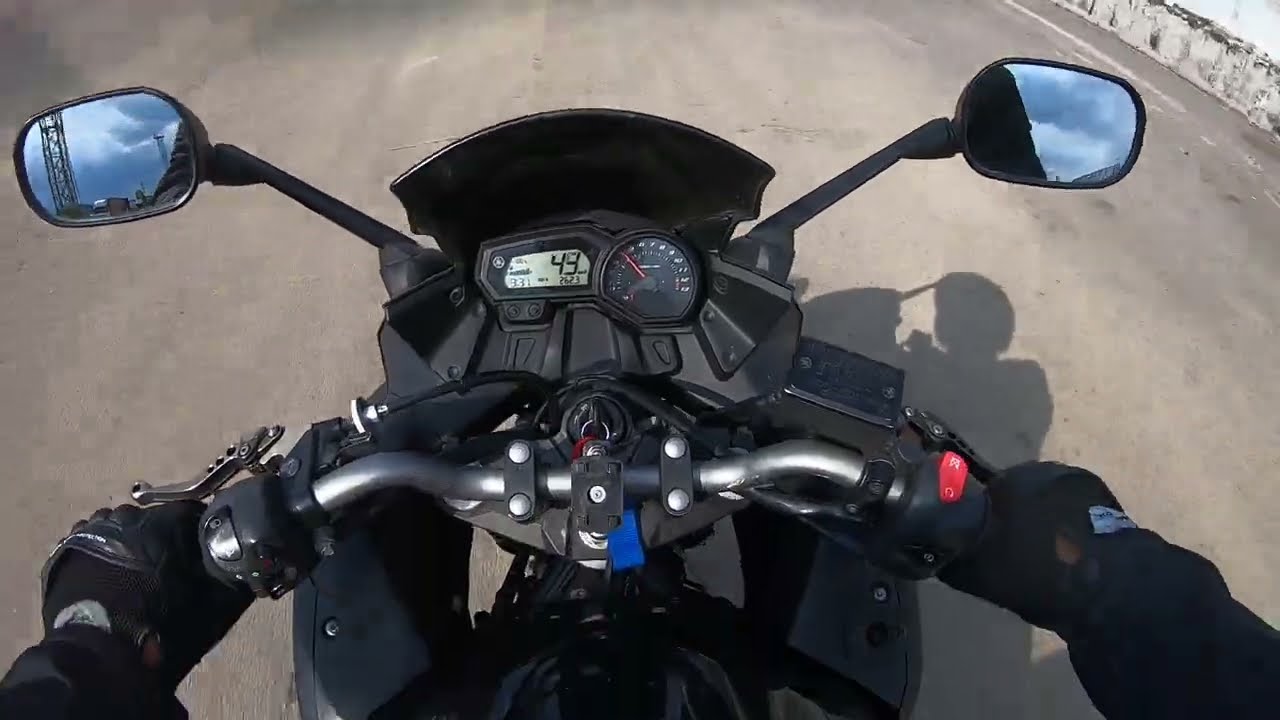The photograph captures a first-person view from a helmet-mounted camera of a rider driving a black motorcycle on a somewhat dusty, grey road. The image predominantly shows the front part of the motorcycle, including the handlebars and dual mirrors. The rider, wearing black gloves and a black long-sleeve jacket, has both hands firmly on the handlebars. The motorcycle’s digital speedometer reads 49, and it is clear that the tachometer needle is positioned towards the left side. The rider is moving under a blue sky dotted with clouds, with the sun positioned behind, casting the rider's shadow forward. In the left mirror, a distant tower can be seen, while the right mirror reflects the sky. Additionally, a red keychain is attached to the motorcycle's key, adding a splash of color to the scene. The time displayed on the speedometer is 13:31.